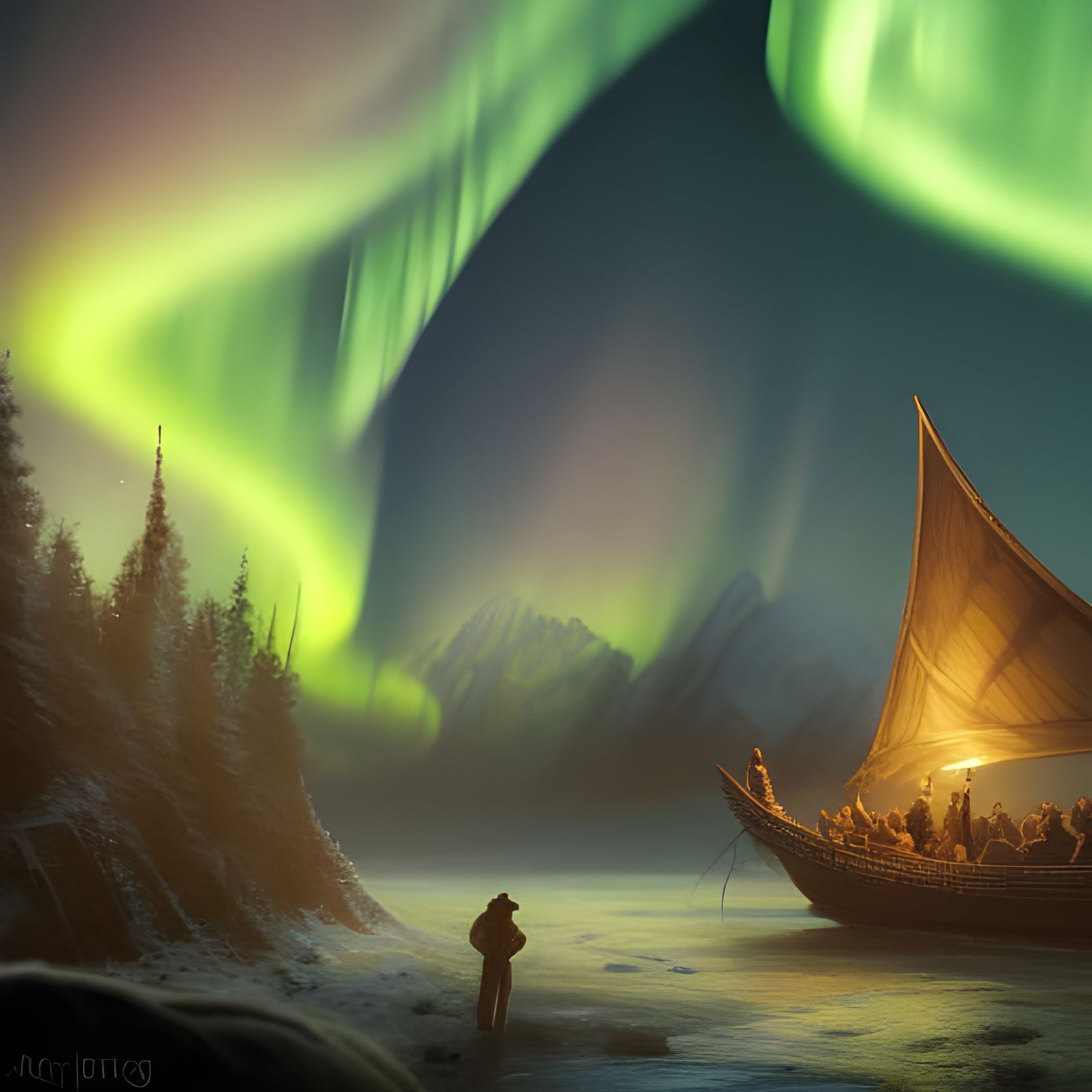The image is a detailed digital illustration depicting a night scene illuminated by the Northern Lights. A vibrant green aurora waves across the dark sky, casting an ethereal glow over the landscape. In the center far distance, majestic mountains rise, partially shrouded by mist or gas. To the left, rocky hills topped with tall pines frame the scene, giving it a rugged, natural beauty.

In the foreground, a lone silhouette of a man stands on the shoreline, his back to the viewer as he gazes towards a large, old-fashioned Viking-style sailboat. The boat is packed with fur-clad passengers, all fixated on the mesmerizing sky. A single torch, held by one of the figures on the boat, emits a dim, flickering light that highlights the icy waters below. The boat appears to be setting sail or perhaps just arriving, its prow facing towards the left.

The artist’s signature can be faintly seen in the bottom left corner, although it is not easily readable. The overall scene captures a moment of solitude, exploration, and wonder amidst a breathtaking natural phenomenon.